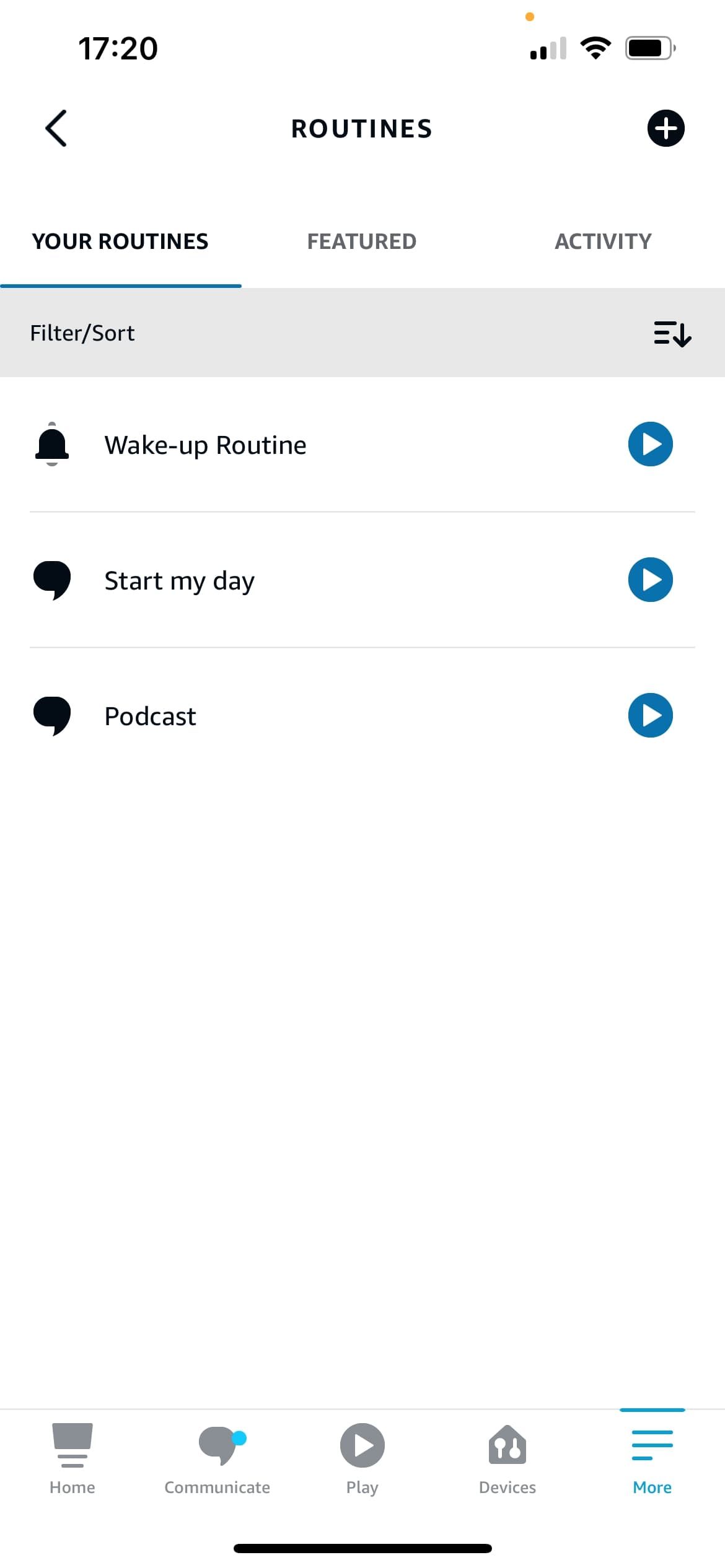The image showcases the interface of a routines management app. At the top, the title "Routines" is prominently displayed. The interface is divided into three primary sections: "Your Routines," "Featured," and "Activity." Currently, the "Your Routines" section is selected. Within this section, three routines are listed: "Wake Up Routine," "Start My Day," and "Podcast." Each of these routines is accompanied by a blue play button featuring a white triangle pointing to the right, hinting at an audio or video function, though it is unclear which.

The "Wake Up Routine" is marked with an icon of an alarm bell, while both "Start My Day" and "Podcast" have speech bubble icons, possibly indicating verbal content.

The app's design is notably minimalistic, with a substantial amount of white space dominating the background and a minimalist aesthetic. At the bottom of the screen, there are five navigation tabs: "Home," "Communicate," "Play," "Devices," and "More." The "Communicate" tab displays a notification indicator, suggesting an unread message or alert.

Overall, the app's layout emphasizes simplicity and user accessibility, focusing on essential functions without overwhelming the user with unnecessary details.